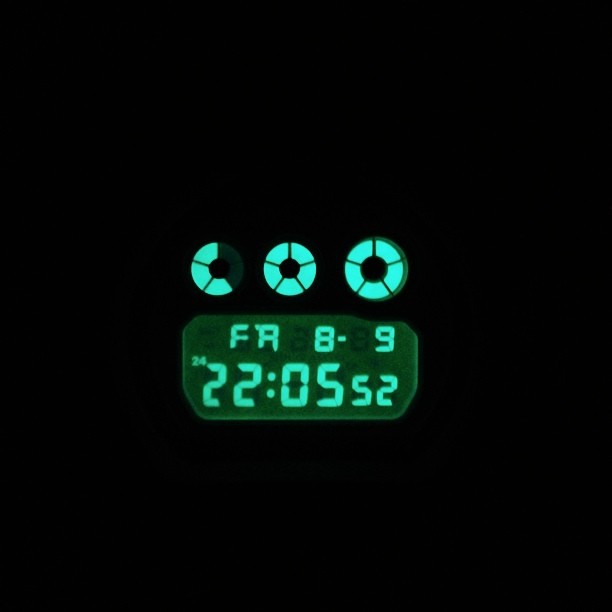In a striking image set against a pitch-black background, only the illuminated portions of a digital watch face are visible. The watch features three circular sections at the top, each divided by five thin plastic spokes, creating a segmented backlight effect. The circles on the far left display only three visible segments, specifically the top left section and two segments below it in a counterclockwise direction. The other two circles are fully illuminated.

The main structure of the watch face is rectangular with slightly rounded edges. It showcases a vibrant green backlight that illuminates the time, depicted in an aqua or lime green color with a hint of blue. The display shows the time in a military format: 22:05:52 (10:05 PM and 52 seconds). To the left of the time, a small number "24" is visible. Above the time, the letters "FA" are positioned just above the "22," and an "8-9" date indicator, representing August 9th, is displayed in the upper right-hand corner.